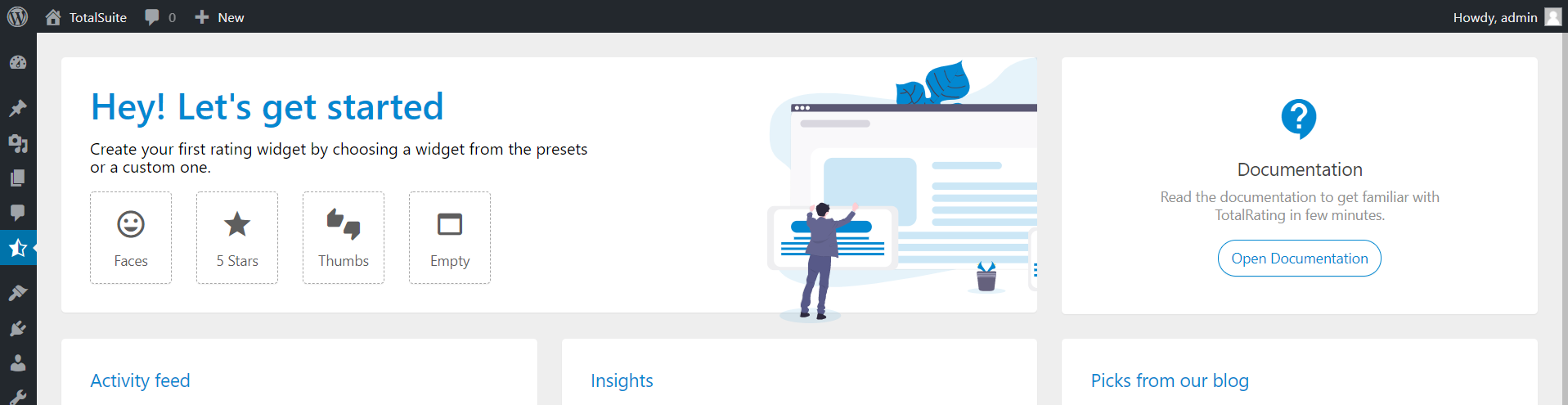The screenshot appears to be of a webpage for "TotalSuite," a WordPress plugin. The website interface features a navigation bar on the left with various icons. These icons include a circle with a "W," an unknown icon, a pin, a stack of two pages, and a text box.

In the center of the page, there is a welcoming message that reads, "Hey, let's get started. Create your first rating widget by choosing a widget from the presets or customize one." Below this message are four vertical rectangles, each representing a different preset widget:
1. **Faces** - Depicted with a happy face icon.
2. **Stars** - Illustrated with a five-star rating.
3. **Thumbs** - Featuring thumbs-up and thumbs-down icons.
4. **Empty** - Shown as a blank page.

On the right side, there is a stylized icon of a cartoon man working on something, represented with colorful lines. Below this icon, there are links for "Documentation," "Activity Feed," "Insights," and "Pick from our Blog." The documentation section encourages users to "Read the documentation to get familiar with total ratings in a few minutes" and provides a link to open the documentation. However, the sections for activity feed, insights, and blog picks are currently empty.

The interface is bordered by a black edge on the left and top sides. At the top right corner, there’s a welcome message that says, "Howdy, Admin," written in white text on the black background.